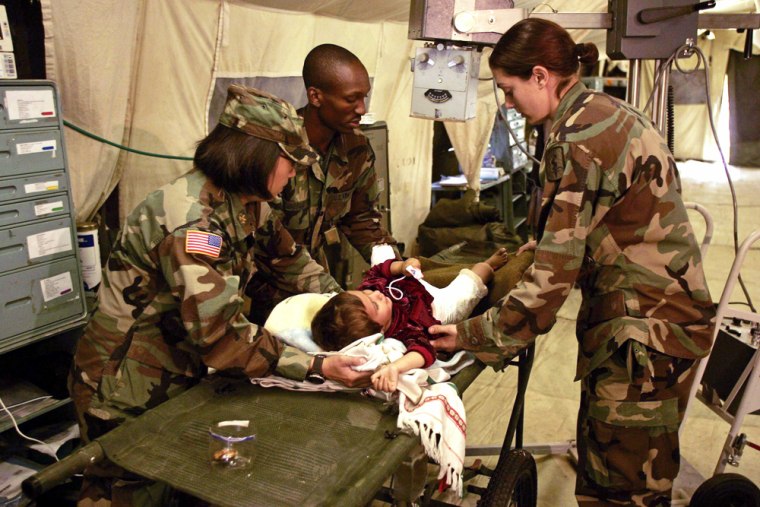The image depicts a scene inside a large military medical tent with white tent walls and plastic or paper-covered floors. At the center, a small child with dark brown hair lies on a green, camo-netted makeshift hospital bed. The child wears a dark red top and white pants and rests on a towel-like pillow or blanket. Attending to the child are three military personnel in camouflage fatigues—two women and one man. The male soldier, who is black, and the two female soldiers, both white with dark hair, stand around the bed. One of the women also wears a matching camo hat. An x-ray machine hovers above the child, indicating some medical examination in progress. Behind them, a gray file cabinet with color-coded cards taped to the drawers—red, blue, yellow, green, and black—can be seen, adding to the makeshift hospital appearance of the tent.